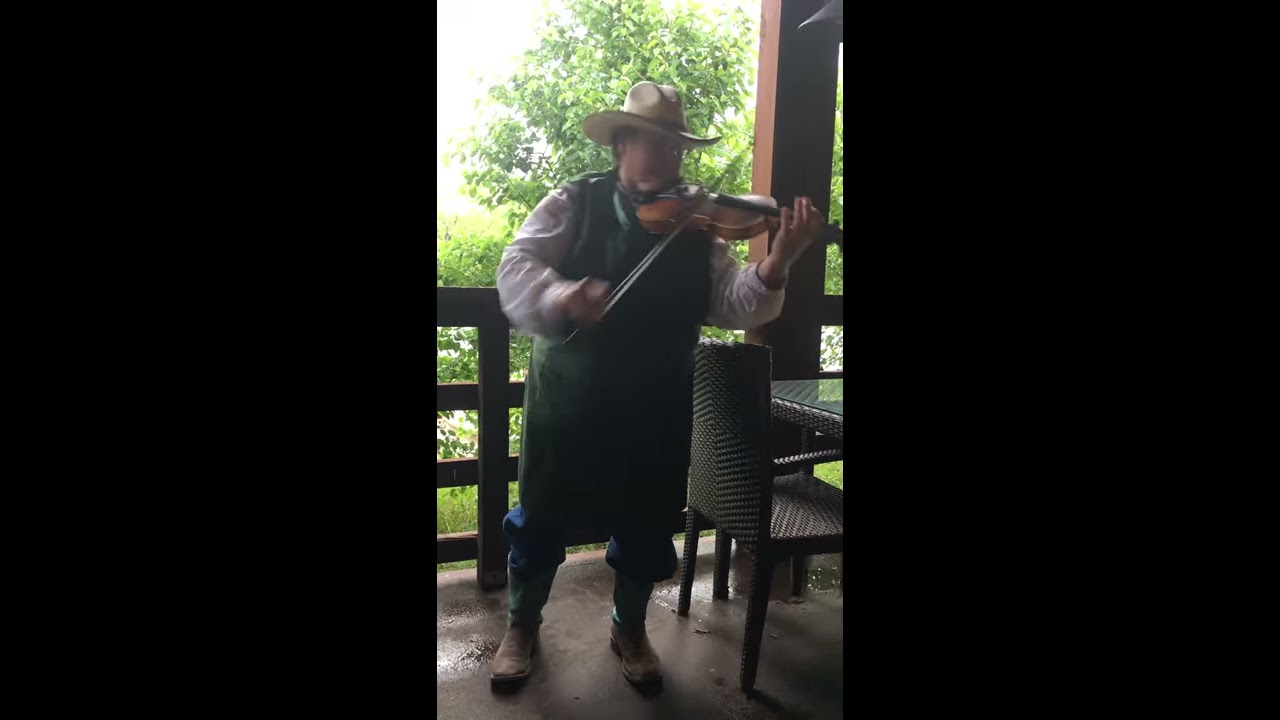The image is vertically partitioned into three equal sections, with the left and right thirds as black borders. The central third showcases a photograph of a man playing a violin or fiddle, his right hand appearing blurry in motion with the bow. The man stands on a cement patio, wearing a pale cowboy hat, a long-sleeved white shirt beneath a sleeveless knee-length green smock, blue jeans, and brown boots. To the right, a large wooden beam and a wicker table with a glass top and a wicker chair pushed underneath are visible. Behind him, a wooden fence, bushes, and a large tree frame the background, with a bright, white, cloudless sky peeking through in the upper left corner.